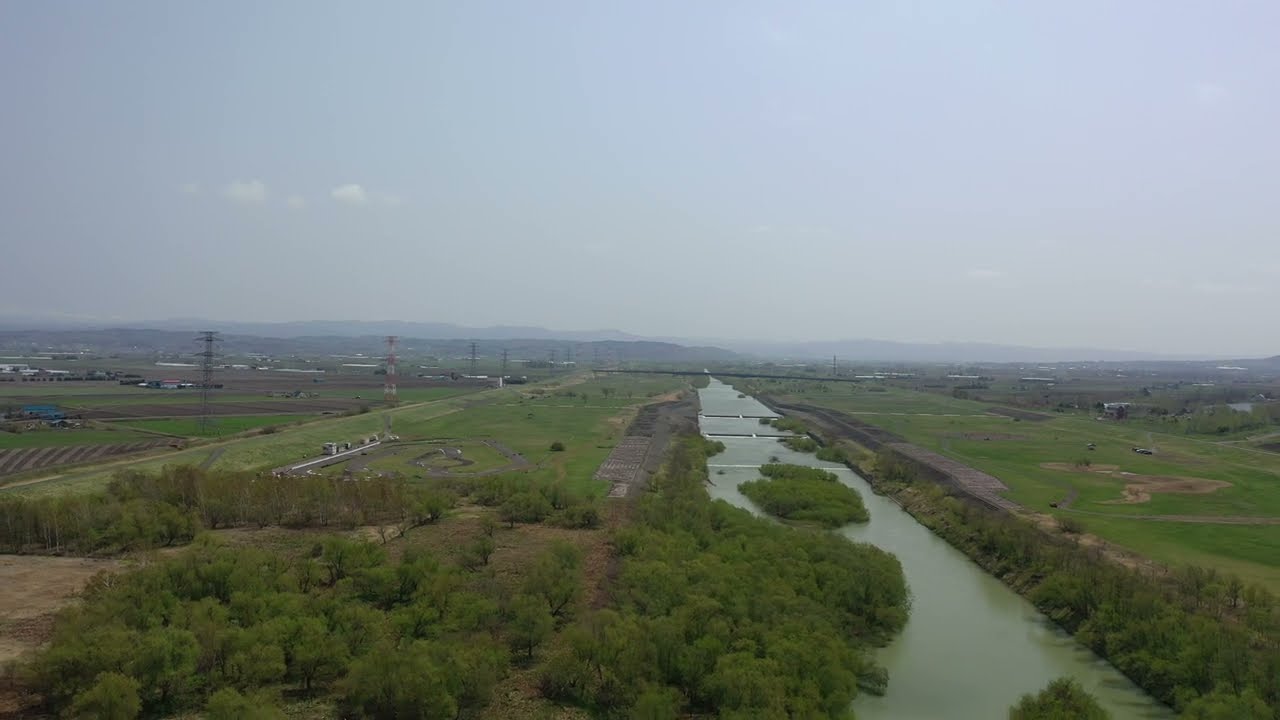This aerial photograph depicts a canal-like waterway running from one side of the image to the other, slightly off-center to the right. The waterway, which appears muddy but is likely clear upon closer inspection, is flanked by various types of shrubbery and bushes along its embankments. A small island of vegetation is also visible within the canal. Surrounding the waterway, there are expansive grassy fields with intermittent patches of brown dirt. 

In the distance, a mountain range with a bluish hue can be seen under a cloudy, hazy sky that gets darker towards the left side of the image. Spotty clouds are present in the top left corner. Power lines run along the left side of the scene, where you can also spot occasional streets and small buildings, with some cars visible as well. The overall landscape appears to be a mixture of farmland and forest, devoid of residential housing for long stretches, contributing to the open and natural feel of the scene.